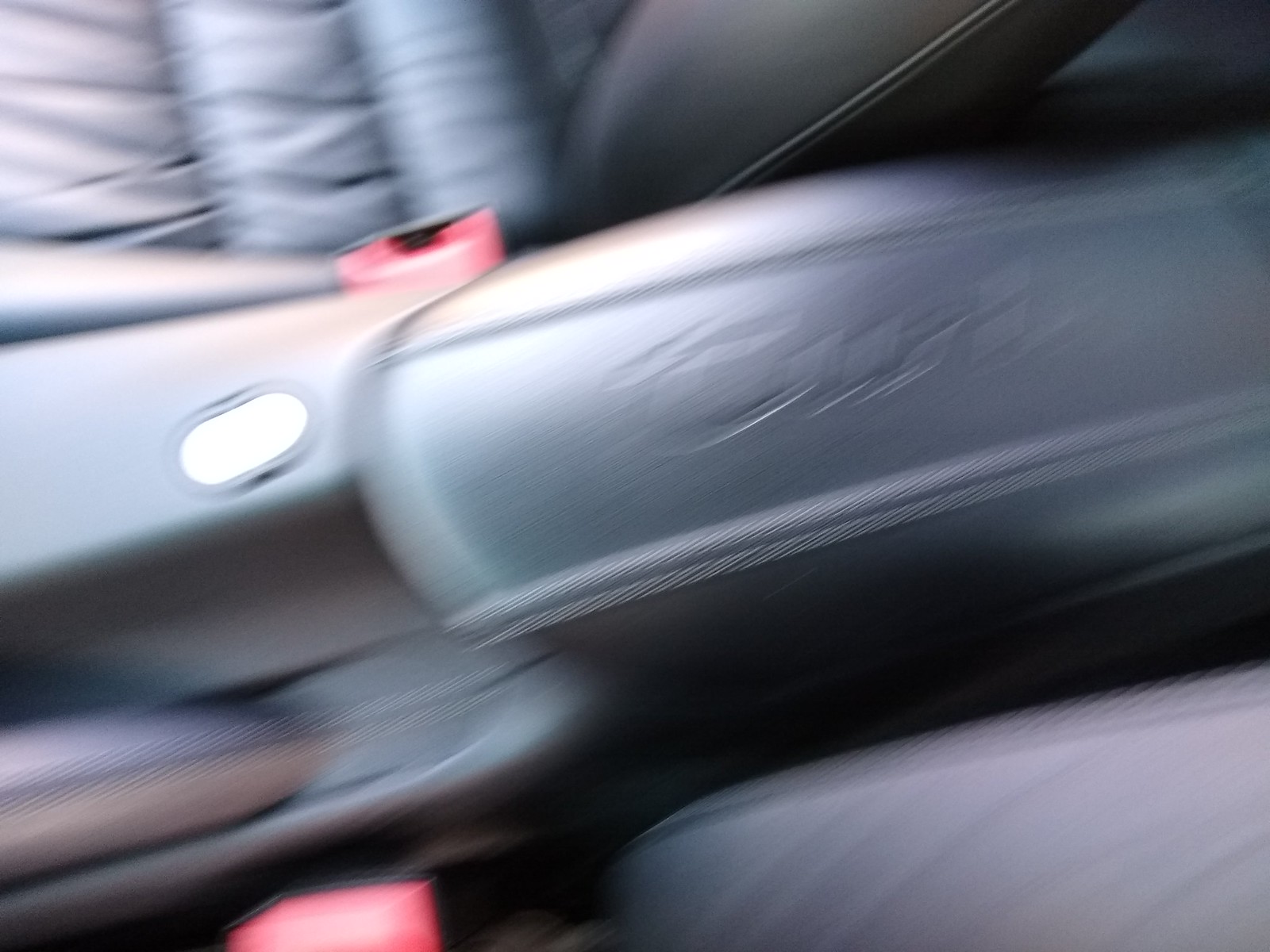This blurry photograph captures the center console of a vehicle's interior. The image, likely taken accidentally, shows a gray-themed interior with leather or leather-like car seats. On the right-hand side, both at the bottom and the top, are the seat belt buckles, positioned parallel to each other. Though there is some writing on the console, it's illegible due to the blurriness. Visible in the frame is a portion of the passenger seat, confirming the gray leather upholstery that permeates the car's design.